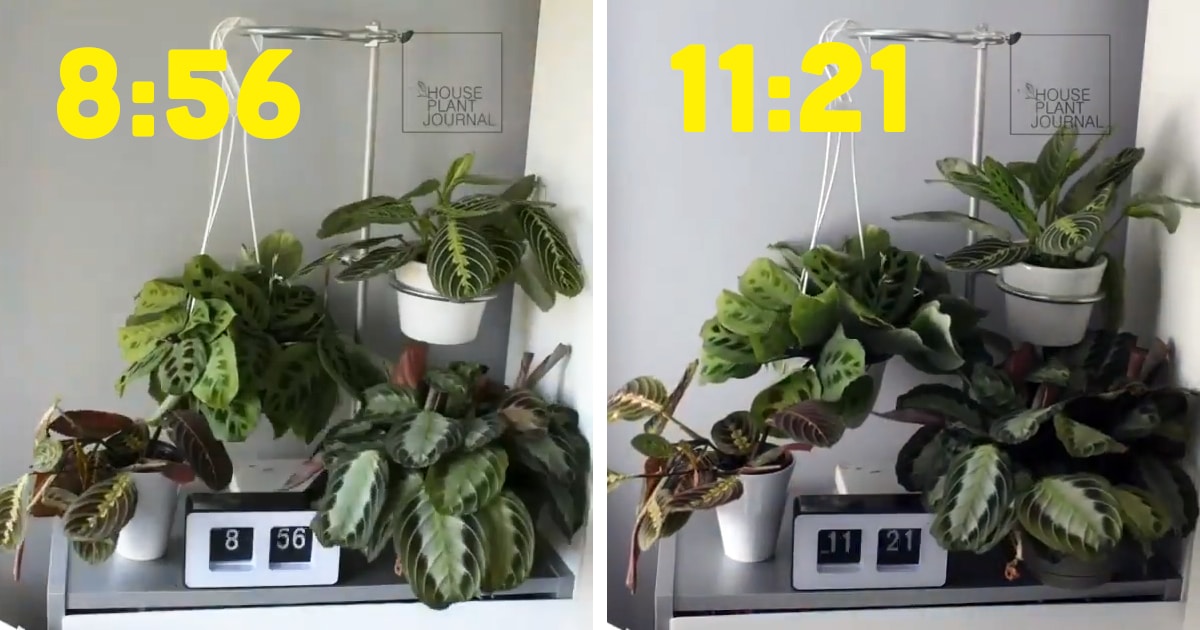The image features a side-by-side comparison of the same scene captured at two different times, as indicated by both the clocks and the time stamps in the top left corners. The left-side photograph is taken at 8:56, displaying a light green wall with "House Plant Journal" written on it. Below this text is a gray table holding several potted plants featuring a variety of leaf shapes and colors, including predominantly green leaves and a striking plant with red leaves. The black and white rectangular digital clock on the table reads 8:56. The right-side photograph captures the same setting at 11:21, with the digital clock and yellow time stamp confirming the time. In this later shot, the plants appear slightly more elevated, suggesting growth or movement. The overall composition remains consistent, emphasizing the subtle changes over the span of a few hours.